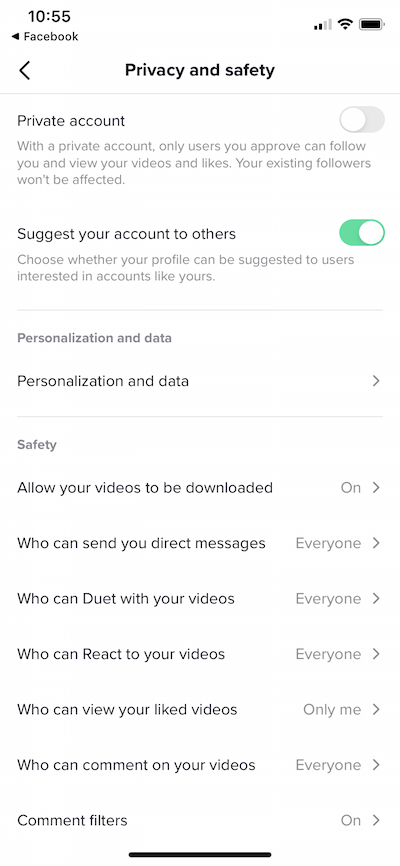The image displays a screenshot taken from a cell phone. The background is predominantly white, and at the top of the screen, the time is shown as "10:55." An arrow icon indicates a navigational option to return to Facebook. To the upper right, there is an icon indicating that the battery is fully charged, represented by a battery symbol filled in black.

Below this, a section titled "Privacy and Settings" is visible, with a left-pointing arrow suggesting navigation. Under this section, the phrase "Private Account" is displayed along with a slider control on the right, which is turned off. 

Further down, there's an option labeled "Suggest Your Account to Others," featuring a green slider with a white ball, indicating that it is turned on. 

Moving further down, another section titled "Personalization and Data" appears, initially in smaller font and then larger with a right-pointing arrow next to it.

Continuing down the screen, "Safety" is listed as a section with several itemized options numbered 1 to 7, including settings such as "Allow your videos to be downloaded" and "Who can send you direct messages: everyone." Additional specific settings about video duet permissions follow in a similar continuation.